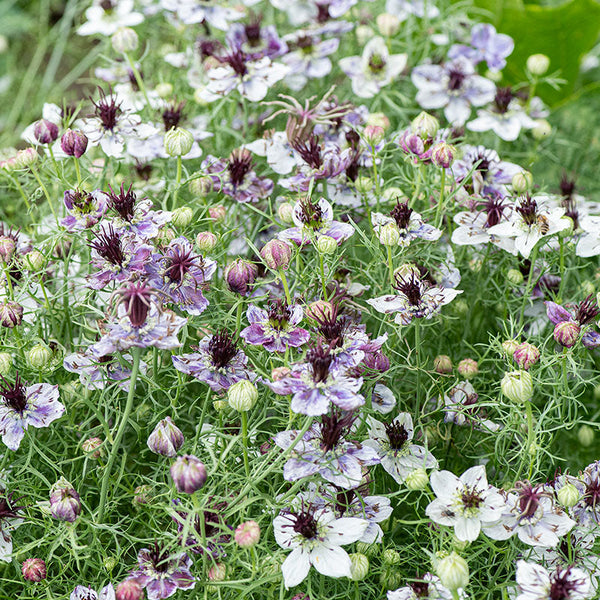The image captures a vibrant and dense display of flowers in a grassy field. Predominantly featuring white and purple flowers, the blossoms vary in color and stage of bloom, with some petals displaying a blend of both hues. The flowers’ centers are generally purple, adding contrast to their white petals. Interspersed among the blooming flowers are roundish bulbs or pods, some showing green veins, awaiting full bloom. The background is primarily green grass with sporadic appearances of brownish spots, particularly toward the back left corner. The overall scene includes a diverse array of flower stems, leaves, and additional plants, with a notable leaf-like object in the back right that is hard to identify. The thin, spindly leaves of the plants create a delicate thread-like appearance throughout the image, contributing to the intricate and rich texture of the floral display.